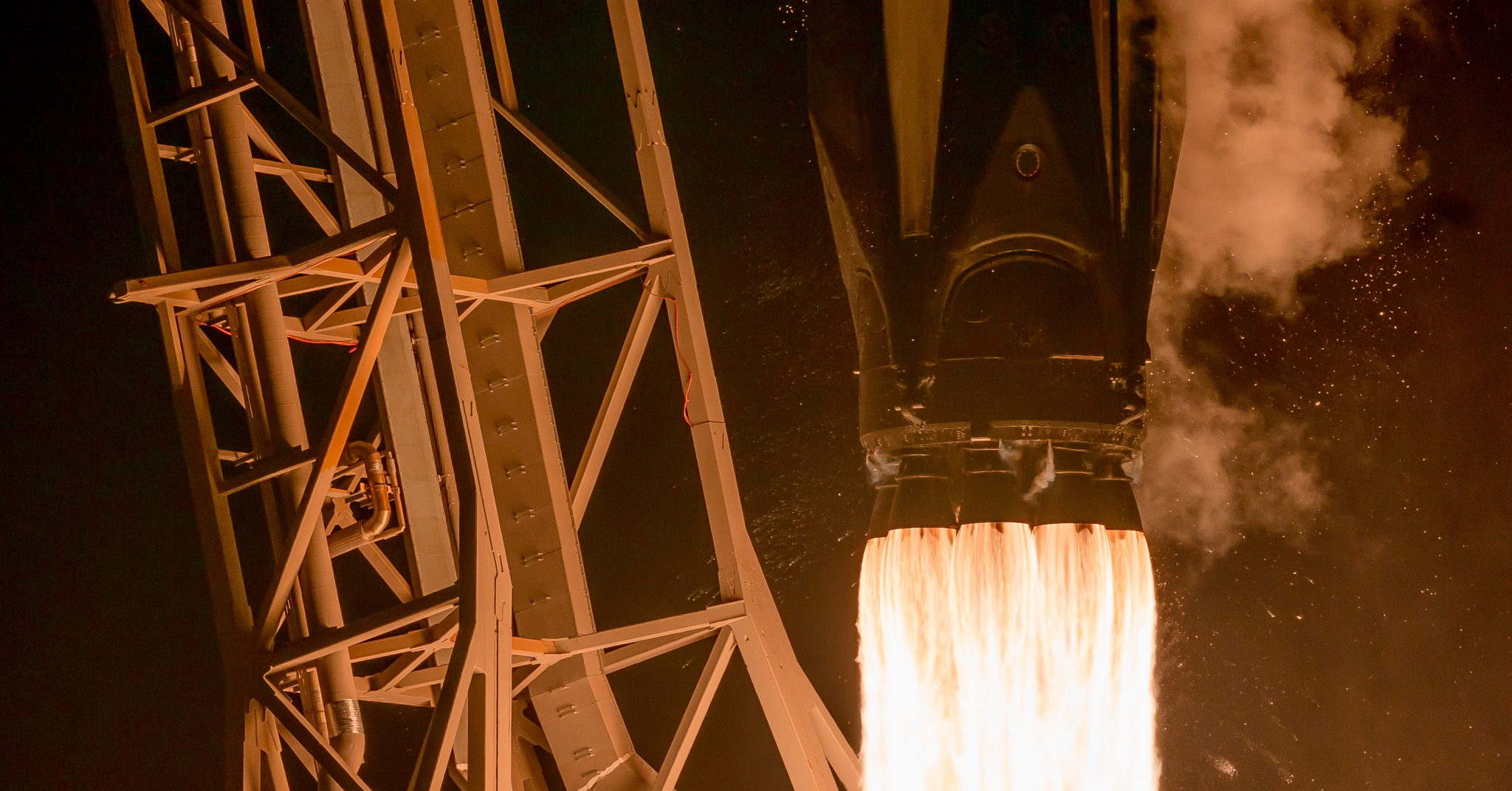The image captures an intense, close-up view of a rocket engine igniting as the rocket blasts off the launch pad at night. Dominating the center is the black body of the rocket, although only the engine section and the plume are visible. From several cone-shaped nozzles at the engine's lower part, bright, predominantly white flames mixed with traces of orange shoot downward. Rising alongside the rocket is a stream of gray-white smoke drifting toward the upper right of the frame. On the left side, a tall, intricate metal scaffolding structure, likely part of the launch system, is visible, composed of bars that intersect at various angles to provide support. This scene is set against a dark night sky, providing a stark contrast that highlights the brilliant flames and intricate details of the launch apparatus.